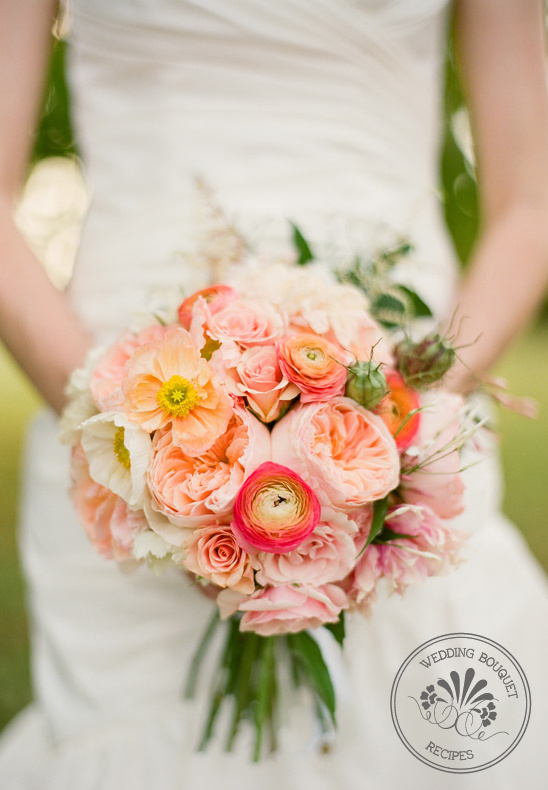This rectangular, real-life photograph serves as an advertisement for "Wedding Bouquet Recipes" and features a sophisticated wedding bouquet as its prime focus. The vibrant bouquet, consisting of tightly packed flowers, primarily showcases pink roses, peach, and salmon-colored blooms, alongside a few reddish or orange flowers with distinctive yellow centers. The bouquet is exquisitely arranged, with approximately 15 different flower bulbs, accentuated by fresh green leaves and stems below. This vivid arrangement is held by a woman in a white, sleeveless bridal dress, her arms and body blurred to emphasize the flowers. The dress, with a flaring bell-like bottom, suggests bridal elegance. The woman's face is not visible, focusing attention solely on the bouquet. In the bottom right corner of the image, a circular stamp in black text reading "Wedding Bouquet Recipes" includes a delicate floral design. Blurred green grass and trees in the background provide a serene, natural setting, enhancing the photograph's emphasis on the bouquet.